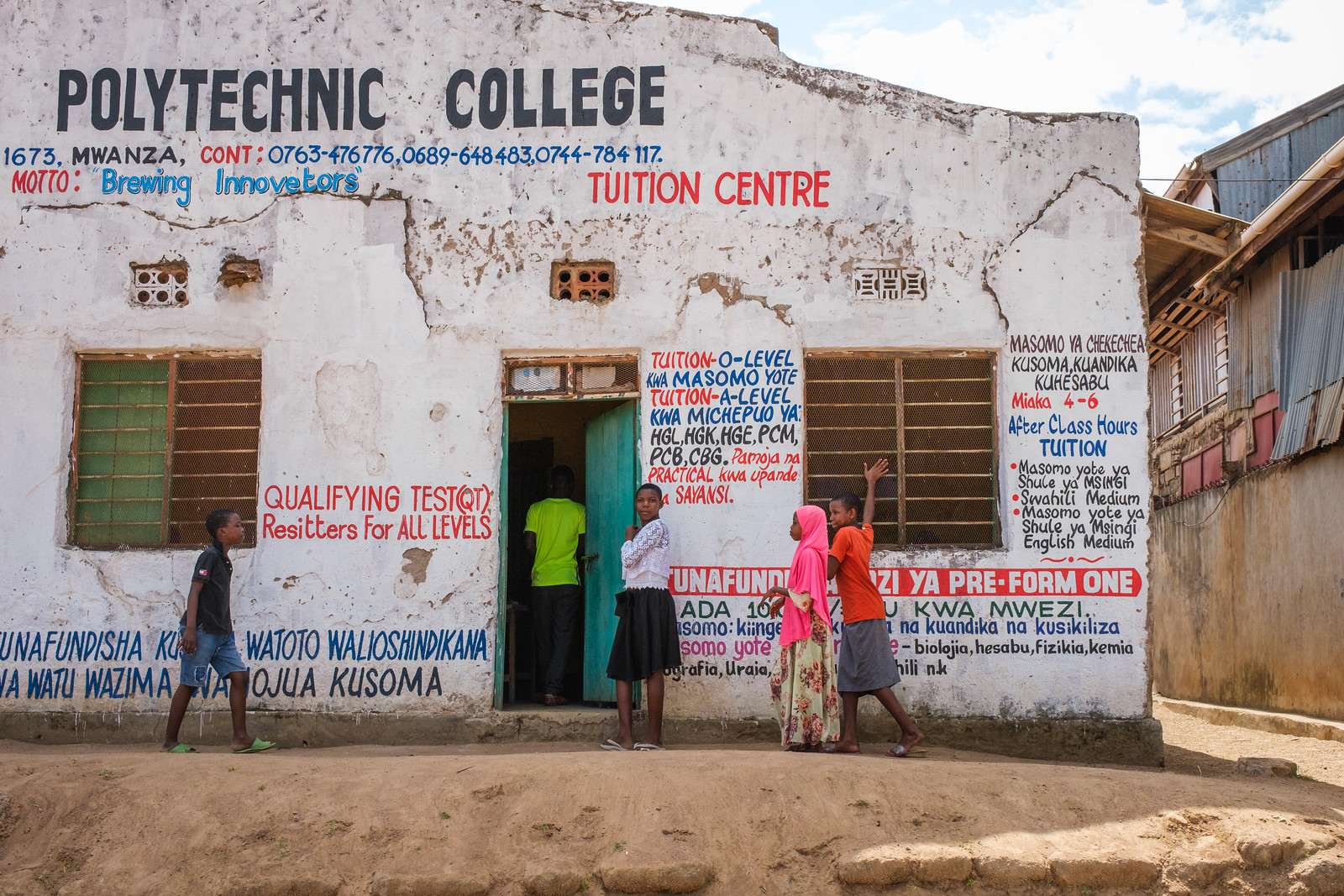This detailed photograph captures a partly cloudy day outside an old, run-down white cement building with significant wear and numerous visible cracks. The building, clearly marked with a black "Polytechnic College" sign at the top and a red "Tuition Center" sign beneath, features various black, red, and blue text detailing the educational services it offers, such as "qualifying tests," "O Level tuition," and "A Level after-hours tuition." The building also has brown windows and additional Spanish writing on the walls.

In front of the building stand four black children: one wears a black shirt with blue jean shorts, a girl is clad in a black skirt with a white top, another child is touching the building while wearing an orange shirt with a gray skirt, and a fifth person, possibly another student, is seen entering through a blue doorway. The image's setting suggests a location in Africa or the Middle East, portraying the polytechnic college as a vital educational facility amidst its dilapidated state.